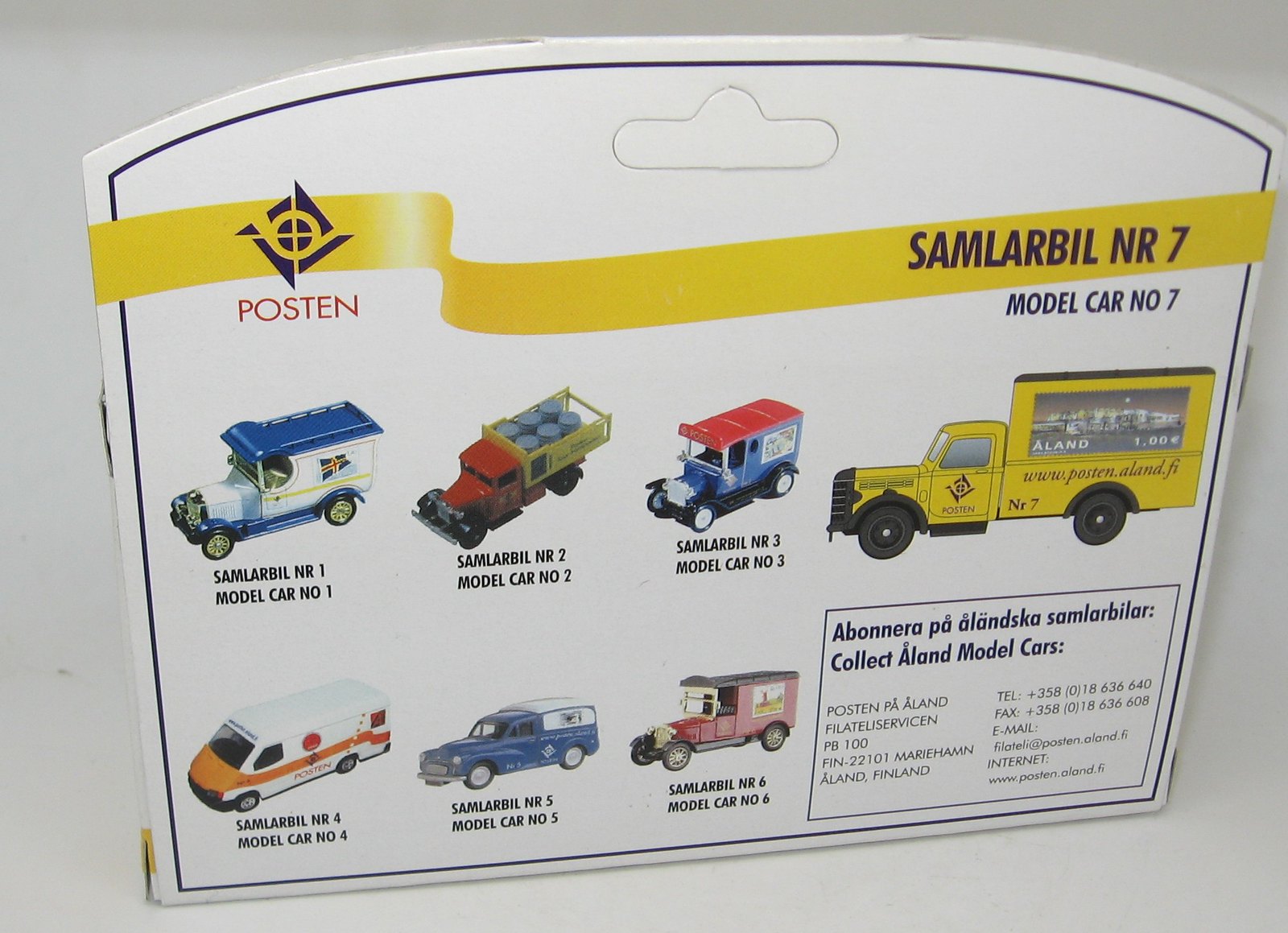The image is of the back of a package for toy trucks, likely from a company named Posten. The package is primarily not in English but mentions Finland, suggesting it might have originated from there. It features a yellow or gold ribbon illustration across the top. On the upper left, there is a logo resembling a quartered square or diamond with a circle in the middle, and beneath it, the word "Posten" in red text. 

The right side of the package reads "Sam Larbill N-R-7," followed by "Model Car Number 7" in English, which refers specifically to a yellow delivery truck depicted prominently on the packaging. The toy line includes seven distinct models of toy trucks. 

In the top row of truck images, from left to right, there is:
1. A white truck with a blue top and blue lower outline.
2. A red truck with a yellow bed carrying six gray cylinders.
3. A blue truck with a white rectangle and some unreadable text, featuring a red roof and black bottom.
4. A side view of a yellow delivery truck.

In the bottom row:
1. A vehicle resembling an ambulance.
2. A blue truck with a white section on its flatbed.
3. A red truck with a black top and bottom, which might look vintage.

The package also includes a rectangle with detailed information about the toy sizes and contact details for the Finnish company.